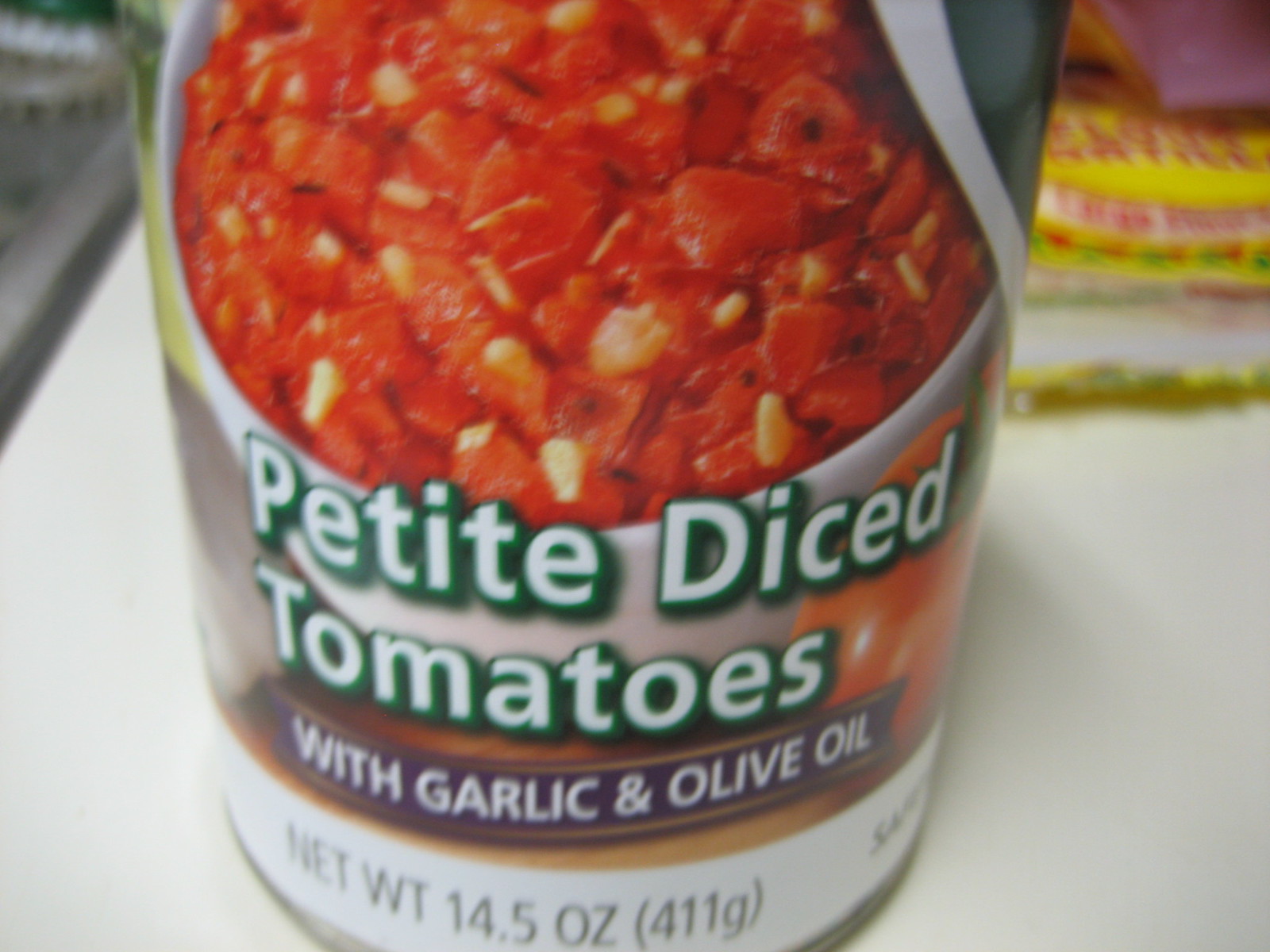The image displays the bottom of a can of petite diced tomatoes immersed in garlic and olive oil. The label features a green background with "Petite Diced Tomatoes" in white font prominently displayed. Beneath this, "With Garlic" is written in white lettering on a purple background. At the very bottom, the net weight is specified as "14.5 ounces (411 grams)" in white with black numbering. The name of the company that produces these tomatoes is not visible. The can is tilted in such a way that it obscures the top, but the primary information about the product is clearly legible.